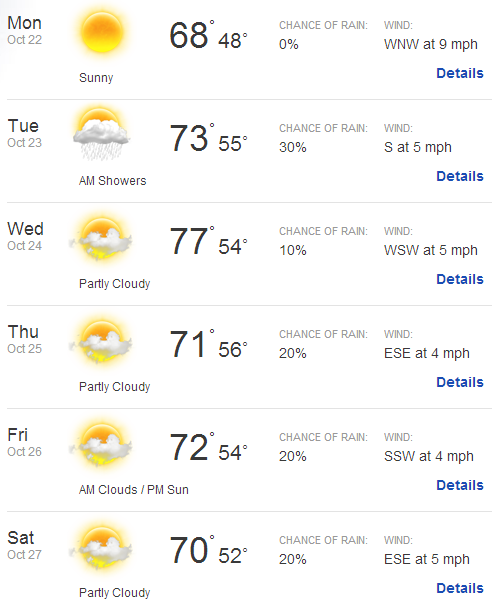A detailed weather forecast is displayed on a weather website, presenting the outlook from Monday, October 22nd, through Saturday, October 27th. Listed vertically, each day of the week is accompanied by an icon depicting the expected weather conditions, followed by a text description:

- **Monday, October 22nd:** Sunny
- **Tuesday, October 23rd:** AM showers and sun
- **Wednesday, October 24th:** Partly cloudy
- **Thursday, October 25th:** Partly cloudy
- **Friday, October 26th:** AM clouds, PM sun
- **Saturday, October 27th:** Partly cloudy

Next to the weather descriptions, the high and low temperatures for each day are provided:

- **Monday:** High of 68°F, Low of 48°F
- **Tuesday:** High of 73°F, Low of 55°F
- **Wednesday:** High of 77°F, Low of 54°F
- **Thursday:** High of 71°F, Low of 56°F
- **Friday:** High of 72°F, Low of 54°F
- **Saturday:** High of 70°F, Low of 52°F

Following the temperatures, the chance of rain is indicated:

- **Monday:** 0%
- **Tuesday:** 30%
- **Wednesday:** 10%
- **Thursday:** 20%
- **Friday:** 20%
- **Saturday:** 20%

The wind speeds for each day are also noted:

- **Monday:** 9 mph
- **Tuesday:** 5 mph
- **Wednesday:** 5 mph
- **Thursday:** 4 mph
- **Friday:** 4 mph
- **Saturday:** 5 mph

Additionally, there is a purple "Details" link beneath the wind speed for each day, suggesting that users can click to access more detailed and specific weather information for that day.